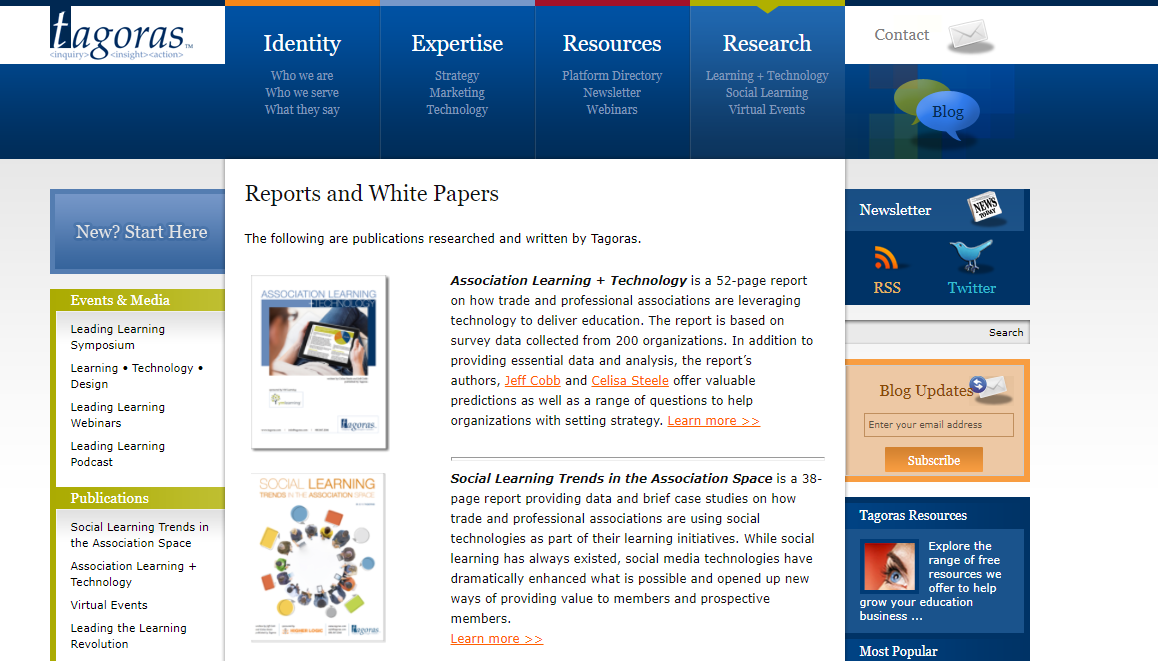The image depicts a detailed layout of a website's homepage. At the top, a series of narrow horizontal lines stretch across the screen, transitioning through various colors: starting from black, then shifting to orange, light blue, red, chartreuse, and finally back to black. Beneath these lines, there is a black banner featuring the text "Tagoras," in white capital letters.

Below the black banner, the rest of the website is set against a blue background. The navigation menu includes links labeled "Identity," "Expertise," "Resources," and "Research." Adjacent to this menu is a contact banner represented by an envelope icon.

Further down, against a blue background with a gray sidebar, there are two thought bubble icons, one of which is blue with the word "Blog" written inside. Slightly below that, in a blue rectangle, the text "NEW! Start Here" is prominently displayed in white font.

Continuing down the page, a green banner appears, listing "Events and Media" and "Publications". Additionally, there is a white text section labeled "Reports & White Papers," accompanied by various detailed paragraphs providing further information on these topics.